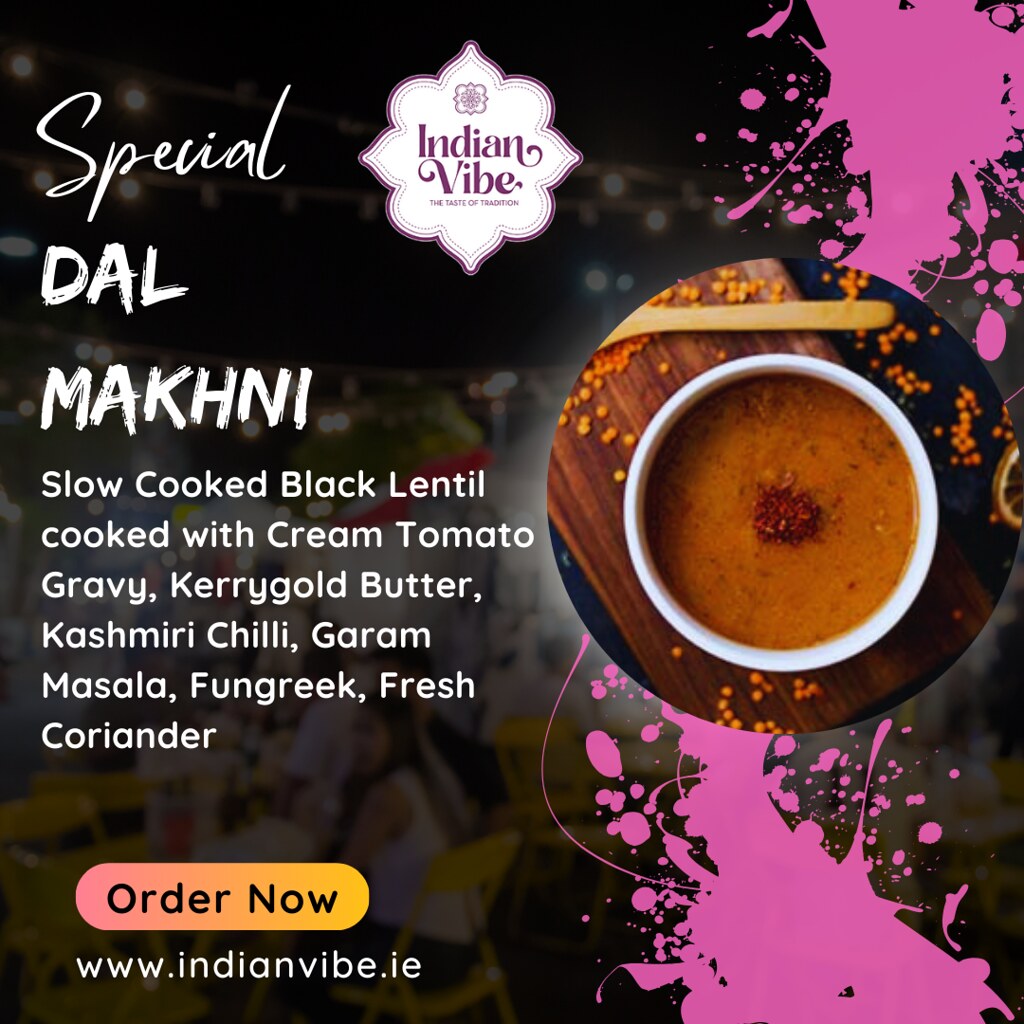The image is a detailed advertisement for an Indian restaurant named "Indian Vibe," showcasing their special dish, Dal Makhani. The backdrop is a dark hue, possibly blue or brown, with faint outlines of people sitting in a restaurant, enhancing its cozy ambiance. A striking feature is the artistic pink paint splatter on the right side, which adds a vibrant touch. The center of the image is dominated by a white, small bowl placed on a brown chopping block, filled with an orangish Dal Makhani, garnished with spices or peppers. The caption, "Special Dal Makhani," is displayed prominently in a distinctive font, differentiating it from the detailed description of the dish, which includes "slow-cooked black lentil cooked with cream tomato gravy, Aguri gold butter, Kashmiri chili, garam masala, fenugreek, and fresh coriander."

At the top of the advertisement, the restaurant's logo is elegantly featured, with "Indian Vibe" in old-timey purple font and the tagline "Taste of Tradition." The bottom of the ad provides a call to action, saying "Order now" with the web address www.indianvibe.ie, inviting viewers to experience this enticing dish.